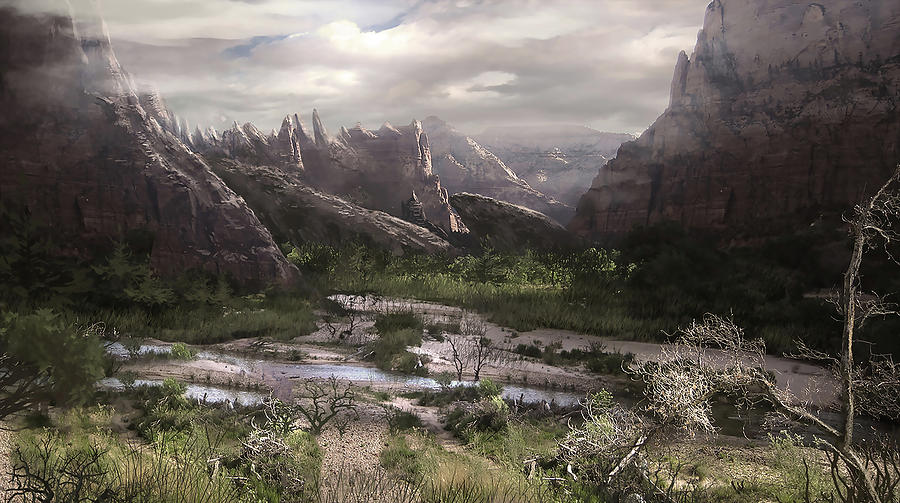The image is a highly realistic digital fantasy landscape featuring jagged, spiky mountain ridges that stretch across both sides of the scene. The mountain peaks, in a dark, maroon-brown and purple hue, create a dramatic backdrop that feels otherworldly. The sky overhead is heavily clouded, with only sparse patches of blue peeking through, suggesting an impending rainstorm. The foreground is a stark contrast—an arid valley scattered with puddles and sections of water, as if rain has recently accumulated in small pools. Amongst the dying grass and plants, which cover the flat terrain, there are a few desolate trees and bushes devoid of leaves, their brown branches stark against the landscape. A narrow creek meanders through the valley, its sandy banks tinged with a reddish hue that mirrors the mountains' colors. The distant end of the valley appears greener, hinting at more verdant areas ahead. The overall atmosphere is dark and brooding, capturing the essence of a fantastical and rugged wilderness.